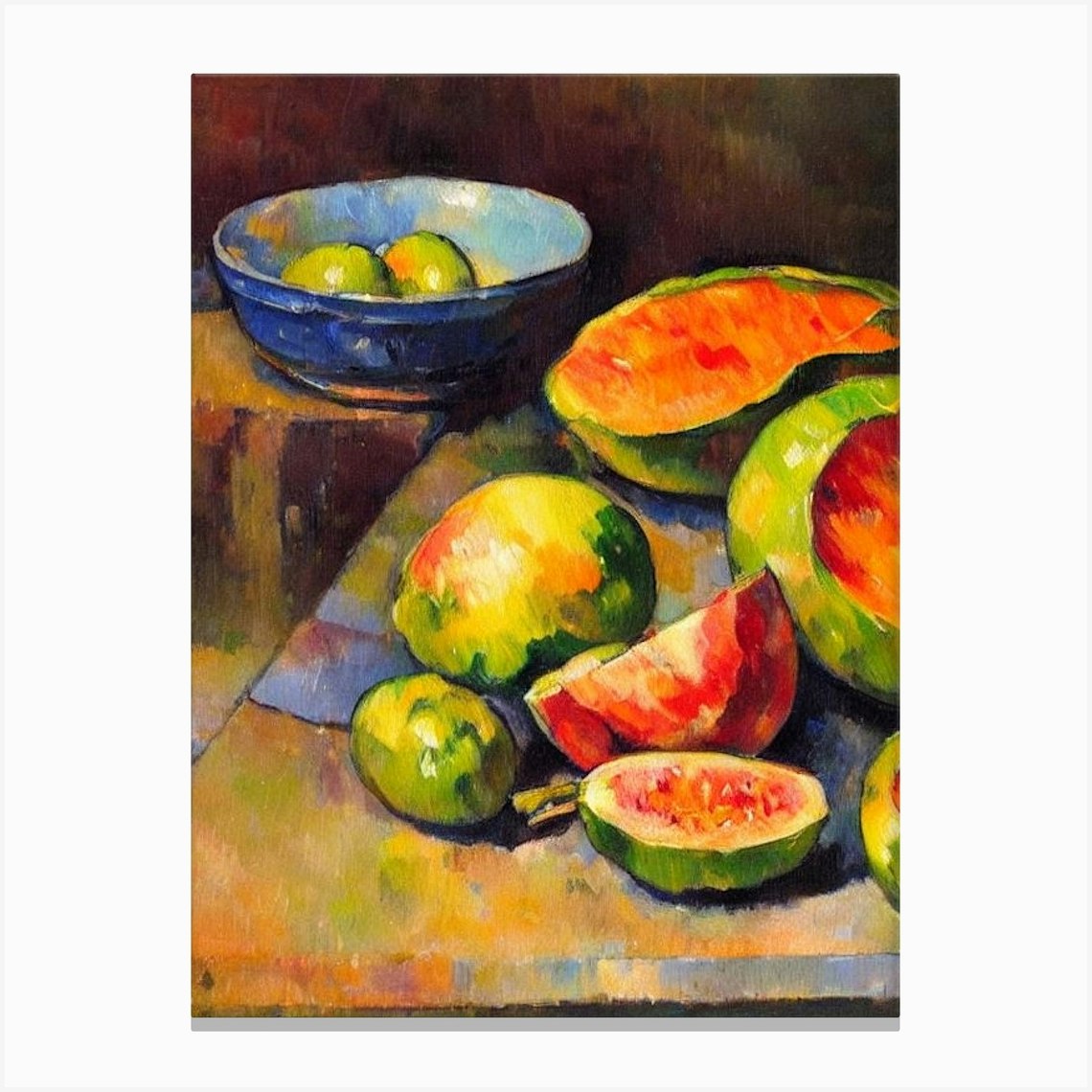This is a vertically aligned rectangular painting with a white background bordered by a faint gray line. The artwork features a still-life composition centered around a collection of fruits. At the top left, there is a blue bowl resting on a counter, containing two pieces of fruit that appear to be green apples. The background in the upper section of the painting is a blend of darker brown tones, suggesting a wall, transitioning to shades of gray and brown near the counter surface. 

The right side of the painting showcases several sliced and whole fruits. The middle and lower portions prominently feature two large chunks of red and green fruit resembling watermelon. Additionally, there's a smaller round green fruit, likely an avocado, and various other fruits with hues of yellow, green, and red. These fruits are arranged on a surface depicted in a mix of gray, blue, yellow, and green tones, creating a contrasting background for the vibrant fruit colors. The detailed portrayal of some cut-open fruits allows the viewer to observe the textures and colors inside, adding a vivid and realistic touch to the composition.